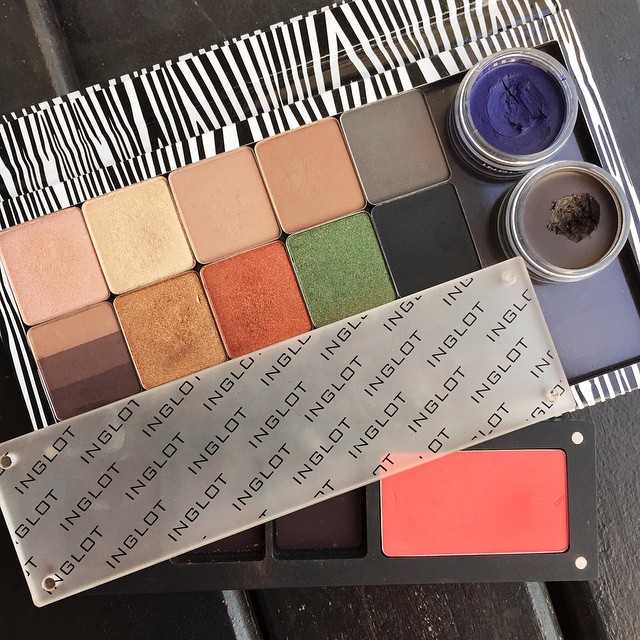The image features a makeup palette with a black and white zebra print border. The palette is laid flat on a table and includes a variety of colors, organized in two rows and five columns, totaling ten square containers. These squares display a range of colors from natural and neutral tones, including flesh-colored shades, pinks, beiges, grays, and browns, to more vibrant ones like green, black, and orange. On the far right, there are two circular pots containing blue and chocolate brown shades, both showing finger marks in their surfaces. The palette has the branding "Inglot" written repeatedly on a frosted panel in the upper left corner, suggesting a folding component. Below this is a secondary section with two square compartments and a larger pink rectangle. The combination of variety in colors and detailed layout suggests it could be used by both artists and makeup aficionados.